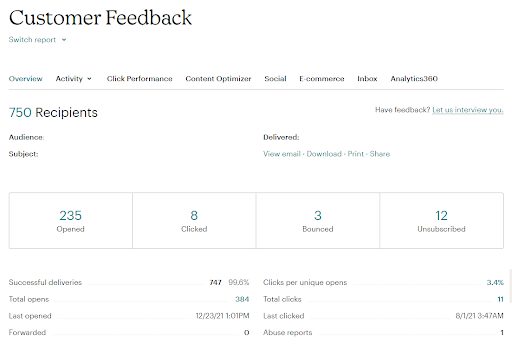This image depicts a detailed web page interface designed to provide feedback and analytics, likely intended for businesses or sellers to review customer interactions and reports. The page features a clean, white background with black text for clarity and readability. Dominating the top portion is a large header that reads "Customer Feedback."

Directly beneath the header is a drop-down menu labeled "Switch Report," allowing users to toggle between different reports. A navigation menu follows, spanning from left to right with options that include: Overview, Activity, Click Performance, Content Optimizer, Social, E-Commerce, Inbox, and Analytics 360.

Further down, a section indicating "750 Recipients" is prominently displayed, followed by a call-to-action on the far right that reads, "Have Feedback? Let Us Interview You." 

Under the "750 Recipients" indicator, the page is divided into sections labeled Audience and Subject. Adjacent to these sections are utility buttons for Delivered, View Email, Download, Print, and Share.

A detailed breakdown of email engagement metrics is displayed below, showing:
- 235 Opened
- 8 Clicked
- 3 Bounced
- 12 Unsubscribed

Additional performance options provided are for:
- Successful Deliveries
- Total Opens
- Last Opened
- Forwarded
- Clicks Per Unique Opens
- Total Clicks
- Last Clicked
- Abuse Reports

This interface offers a comprehensive overview of customer email interaction and performance metrics, essential for data-driven decision-making.